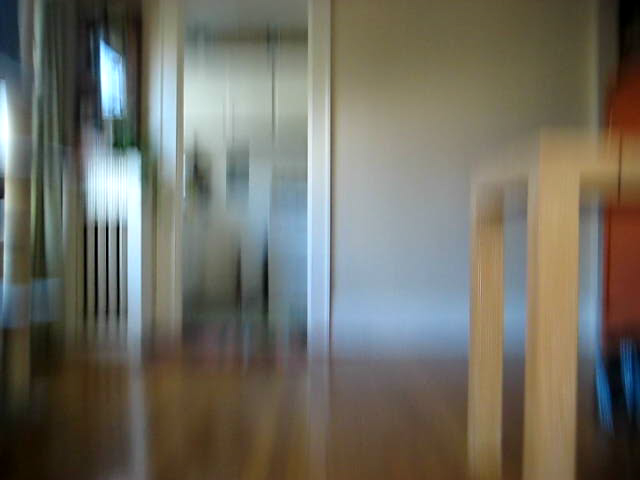The image is a blurry, motion-captured shot of what seems to be a living room interior. On the left side, long window curtains in a light brown color with white, sheer stripes partially obscure a small, brightly lit window. In the center, there is a doorway leading into a white-colored kitchen where upper wall-mounted cupboards can be faintly discerned. The floor throughout the scene appears to be wooden with a brown hue. On the right side of the image, partially visible, is the light brown, wooden leg and edge of a table.